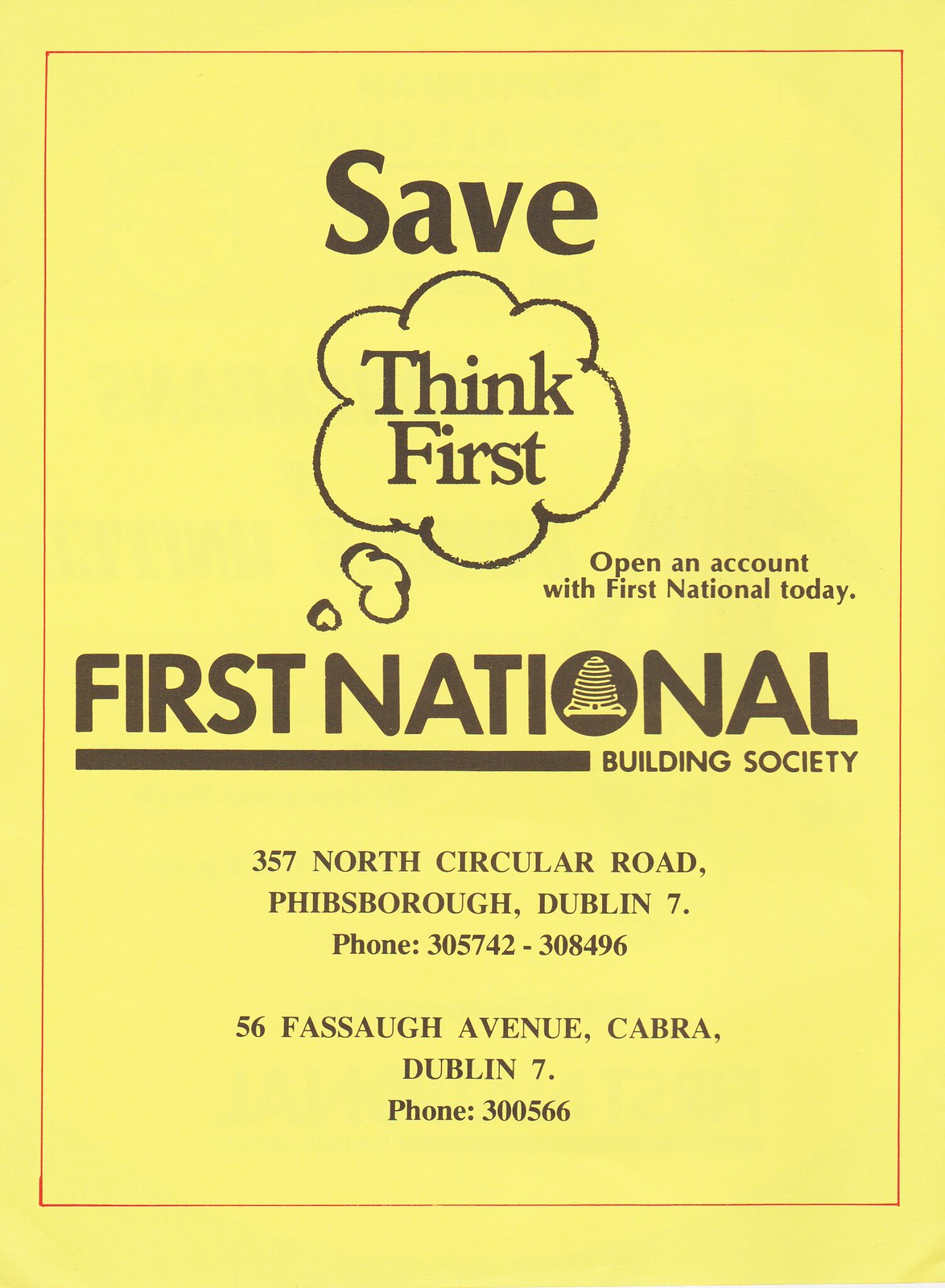This vertically oriented advertisement for the First National Building Society features a yellow background with a reddish border and brownish black text. Prominently displayed in the center is the phrase "Save, think first" enclosed in a thought bubble. Below the thought bubble, the text reads "Open an account with First National today." The ad includes two addresses: 357 North Circular Road, Phibsboro, Dublin 7, with the phone number 305-742-308-496, and 56 Fossil Avenue, Cabra, Dublin 7, with the phone number 300-566.